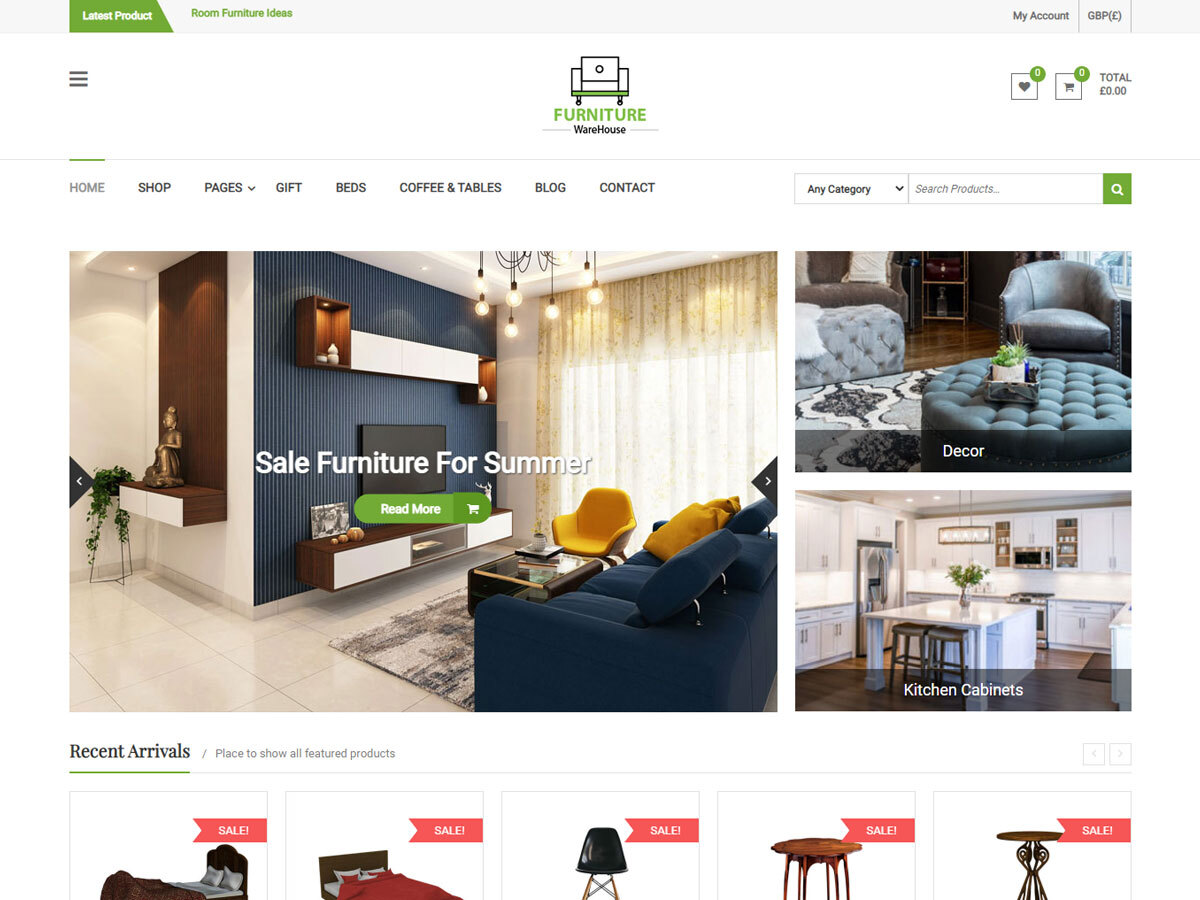The landing page of the Furniture Warehouse online store is meticulously designed with user navigation in mind. 

At the very top, a light gray stripe spans across the page, featuring a green field with white text that reads "Latest Product." Adjacent to this, darker text against the gray stripe announces "Room Furniture Ideas." On the far right side of this stripe, additional links labeled "My Account" and "OVP" are prominently displayed.

Directly below this stripe is the main header showcasing the Furniture Warehouse logo. A hamburger menu is neatly positioned on the far left side for easy navigation. Towards the far right, users can find icons to mark their liked items, a shopping cart, and a total tracker to monitor their cart's total value.

Following the header, the page displays a visually captivating group of photos. One of these images promotes a summer sale with the text "Sale Furniture for Summer," inviting visitors to "Read More." This image depicts a stylish living room adorned with shelves, a mirror, a console, and a tile floor. To its right, another photo showcases a cozy living room arrangement complete with chairs and an ottoman, enhancing the inviting atmosphere. Below these, an image highlights pristine white kitchen cabinets, capturing a sleek and modern kitchen setup.

This composition not only provides a clear and user-friendly layout but also highlights the diverse range of products available, enticing visitors to explore further.